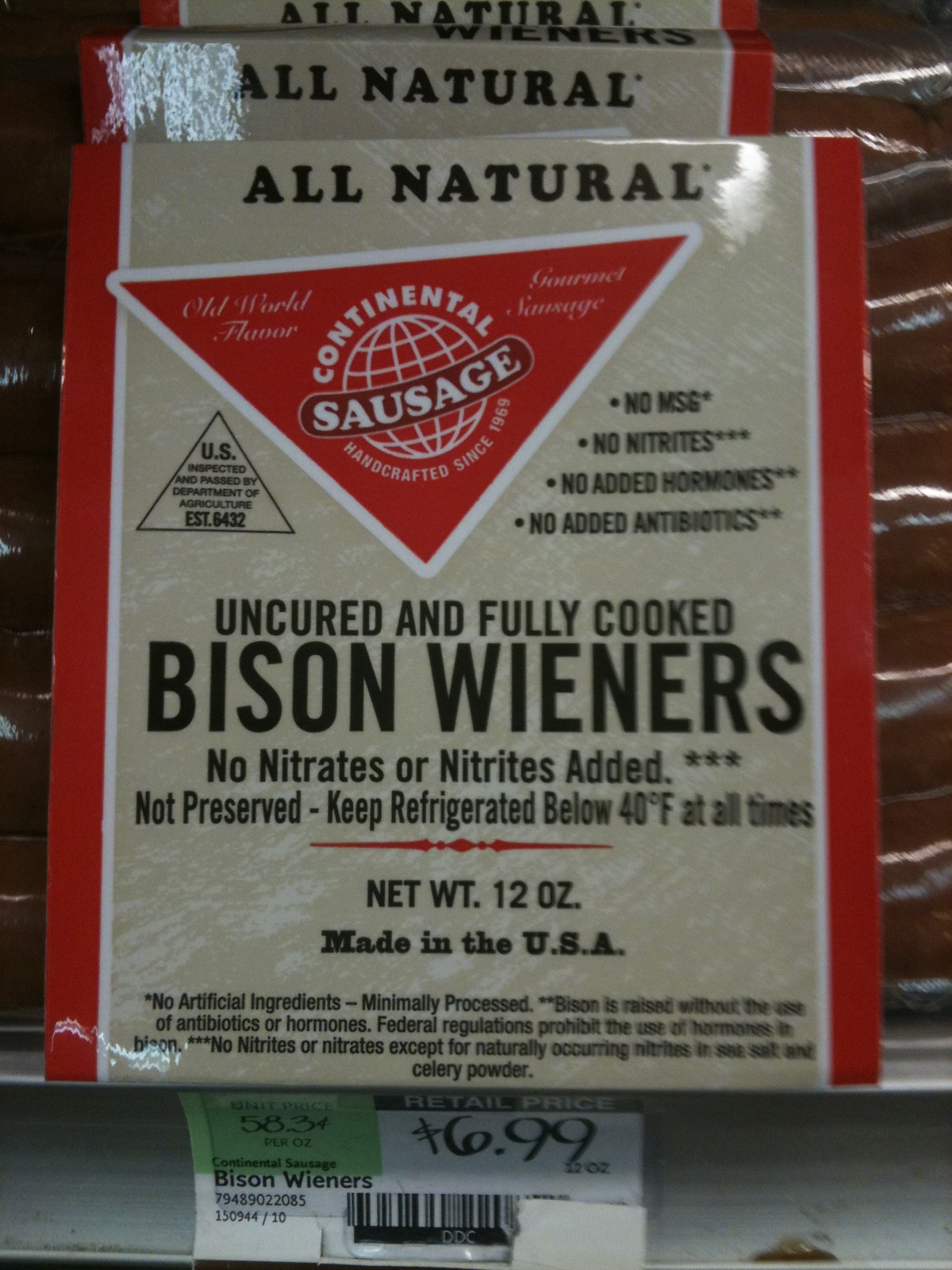A detailed sign on a package of bison wieners reads: "All natural, continental sausage, uncured and fully cooked bison wieners. No nitrates or nitrites added, not preserved. Keep refrigerated below 40°F at all times. 12 ounces, made in the USA. $6.99 per 12 ounces." The packaging is a tannish white color, featuring a red line on one side and a red triangle in the top corner that displays the "Continental Sausage" brand name. Positioned below, a white sticker indicates the price, "$6.99," and identifies the product as "bison wieners." Additionally, a small green sticker specifies the unit price as "58.3 cents per ounce."